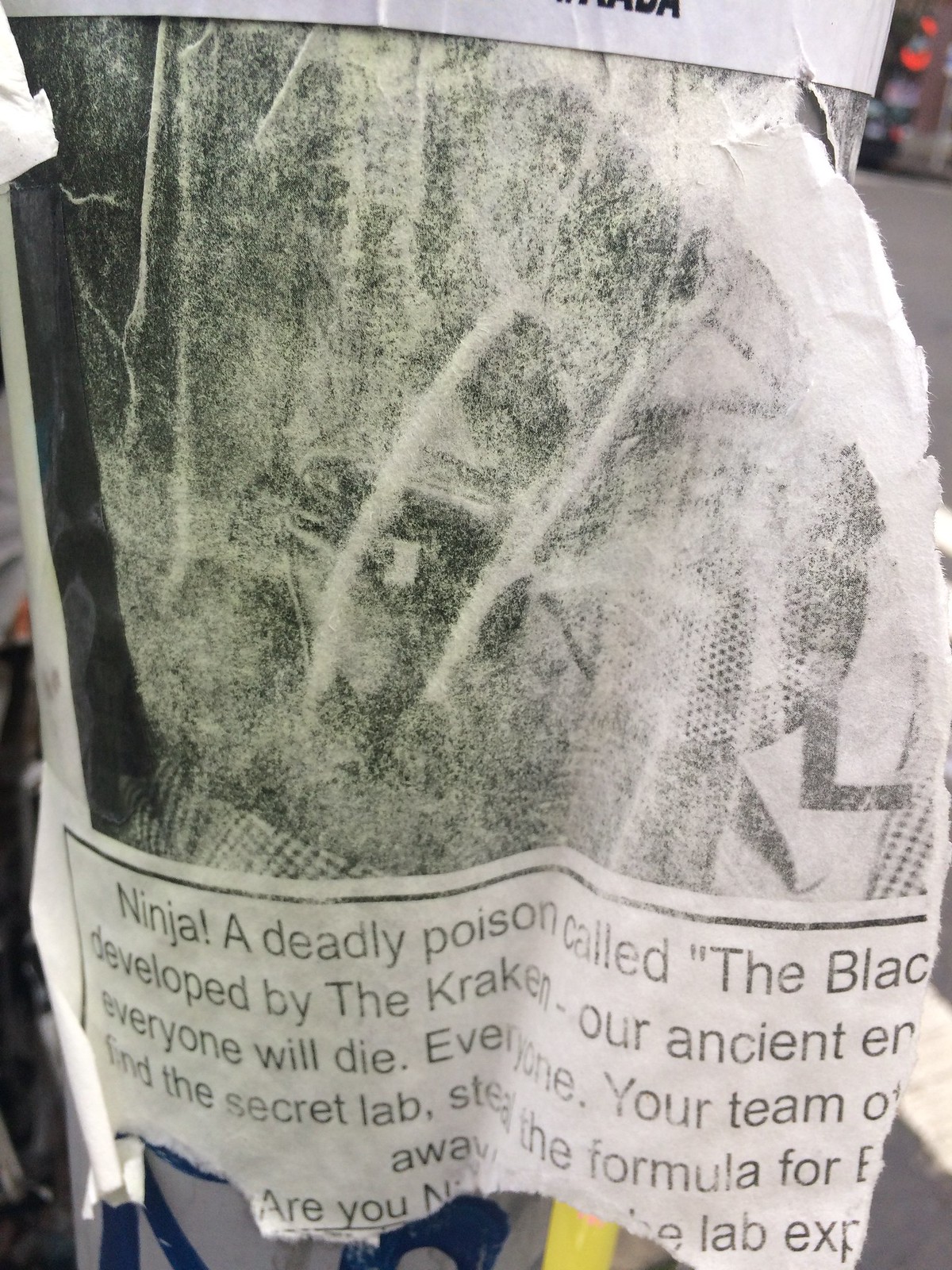The image depicts a significantly degraded and frayed piece of paper wrapped around a city light pole, held in place with tape. Much of the paper is destroyed, but remnants of black ink text are still visible. The visible text reads, "Ninja!" followed by, "A deadly poison called the Black..." though the last part of the word "Black" is cut off. It further mentions the poison being "developed by the Kraken, our ancient..." with subsequent text being unclear, possibly indicating an "enemy." Below, in fragmented and faded print, there's a dire warning that "everyone will die," and an instruction to "find the secret lab, steal the formula for..." with the remainder being illegible. The scene includes a background of a sidewalk made of gray pavement and a distant storefront illuminated by neon lights, including noticeable red and yellow hues, suggesting an urban setting for this mysterious and cryptic message.